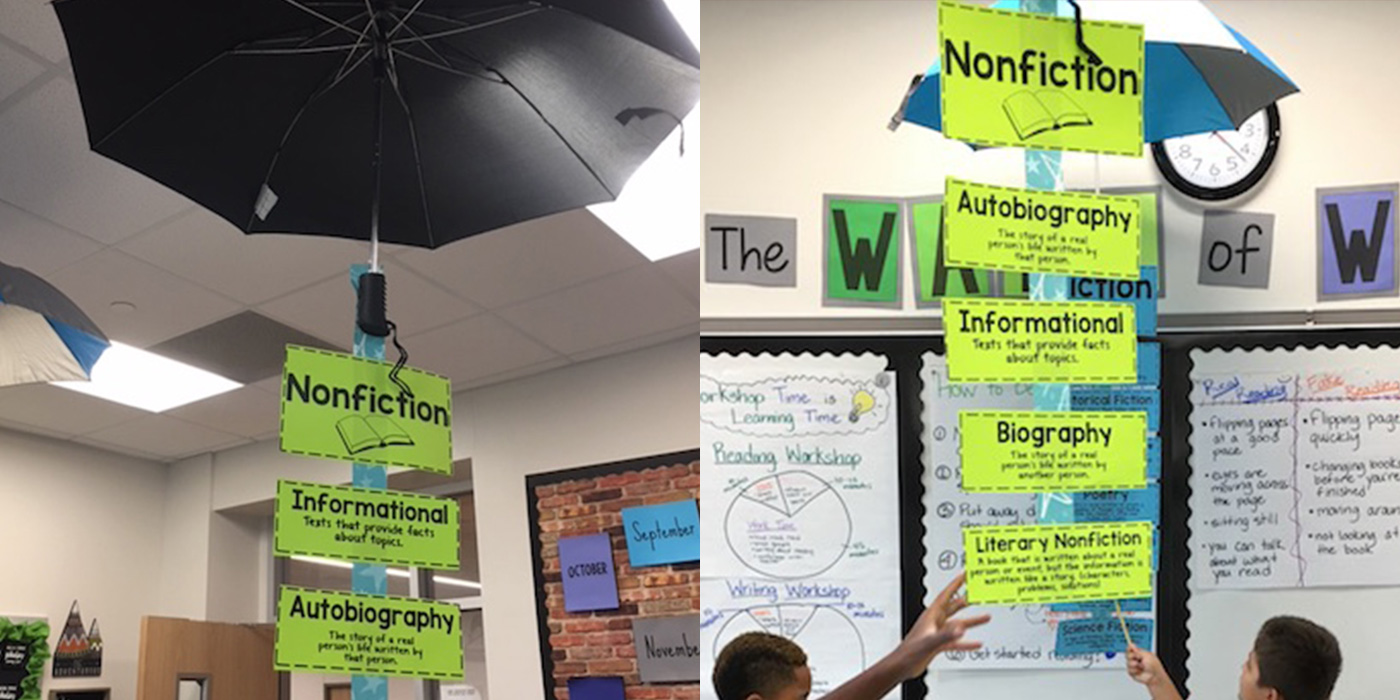The image, likely intended for a school website, comprises two side-by-side photos taken inside an elementary or middle school classroom. Both photos prominently feature classroom decorations and educational material. 

In the left photo, there is a black umbrella suspended from the ceiling with a blue ribbon hanging from it. Attached to the ribbon are several neon green signs with black lettering, listing different types of books: “Nonfiction,” “Informational,” and “Autobiography.” The photo, taken from a low angle, also shows the white, standard-tile ceiling with halogen lighting and a distant view of the classroom door and bulletin board against the white walls.

The right photo, with a similar low perspective, features a blue and white (or gray) umbrella with blue signs hanging from it, partially obscured by more neon green signs displaying: “Nonfiction,” “Autobiography,” “Informational,” “Biography,” and “Literary Nonfiction.” In the background, there’s a clock on the wall and several whiteboards bordered in black wavy trim. These whiteboards display detailed information pertinent to a reading workshop, written in black, blue, and green markers. Two young children are pointing at the bottom neon green sign, enhancing the interactive and engaging atmosphere of the classroom. The overall setting is bright and educational, emphasizing the emphasis on different genres of books and the active learning environment.